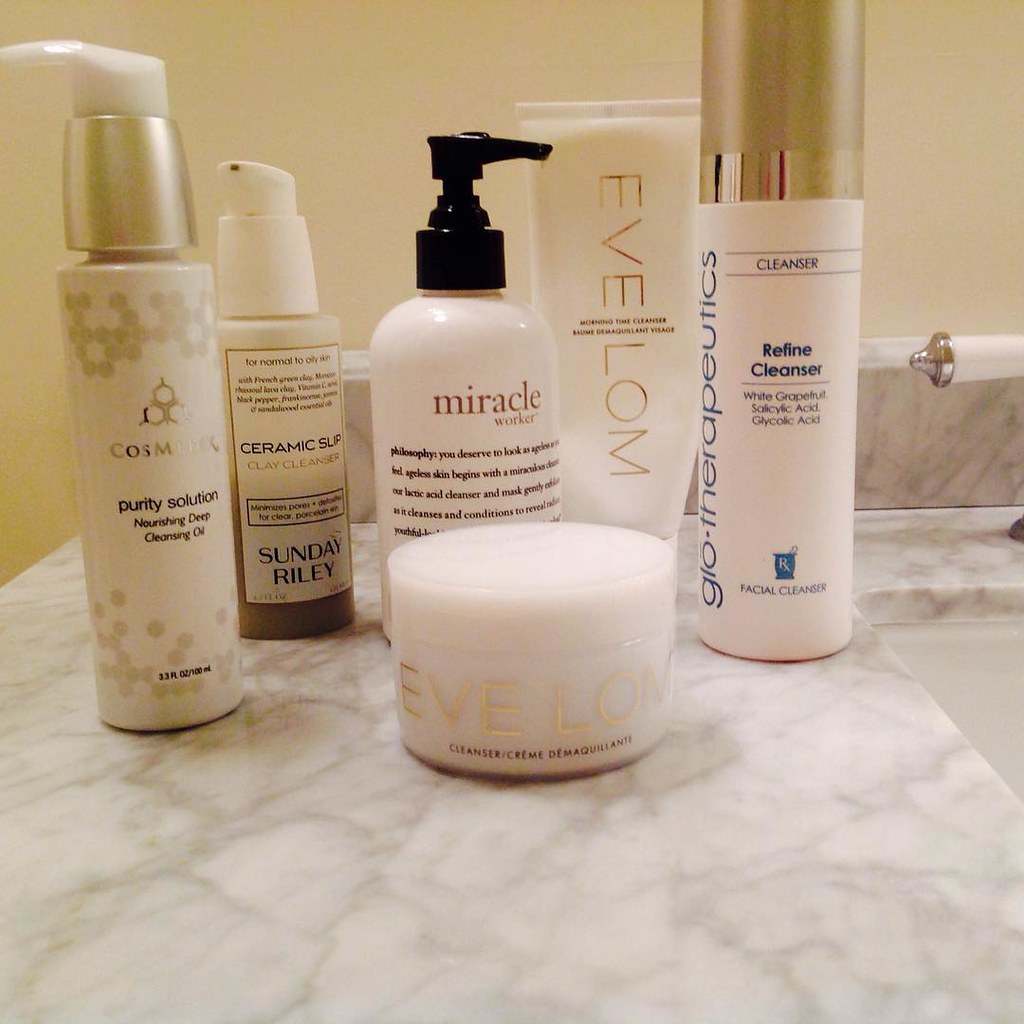The bathroom counter showcases an elegant design with white marble accented by subtle gray veining. On the right side of the image, a white ceramic sink basin is partially visible, featuring a silver metal lever, likely part of the faucet. The background reveals a tan-colored wall, complementing the countertop’s pristine aesthetic. 

On the counter, various beauty products are neatly arranged. These include:

- A white cylindrical container with a gold lid labeled "Glow Therapeutics Cleanser," detailing its contents as "Refined Cleanser, White Grapefruit, Salicylic Acid, and Glycolic Acid Facial Cleanser."
- Two Eve Lom products: one labeled "Morning Time Cleanser" and another smaller container marked as "Cleanser Cream," both featuring white lids.
- A pump-style hand soap bearing the label "Miracle Worker," with a black pump and white bottle.
- A tan bottle with a white label demonstrating blue print, identified as "Ceramic Slip Clay Cleanser" by Sunday Riley, suitable for normal to oily skin and capped with a white pump.
- Lastly, a tan and gold cylindrical container with a gold lid and white pump, named "Purity Solution."

Every item adds to the sophisticated yet functional ambiance of this well-organized bathroom counter.